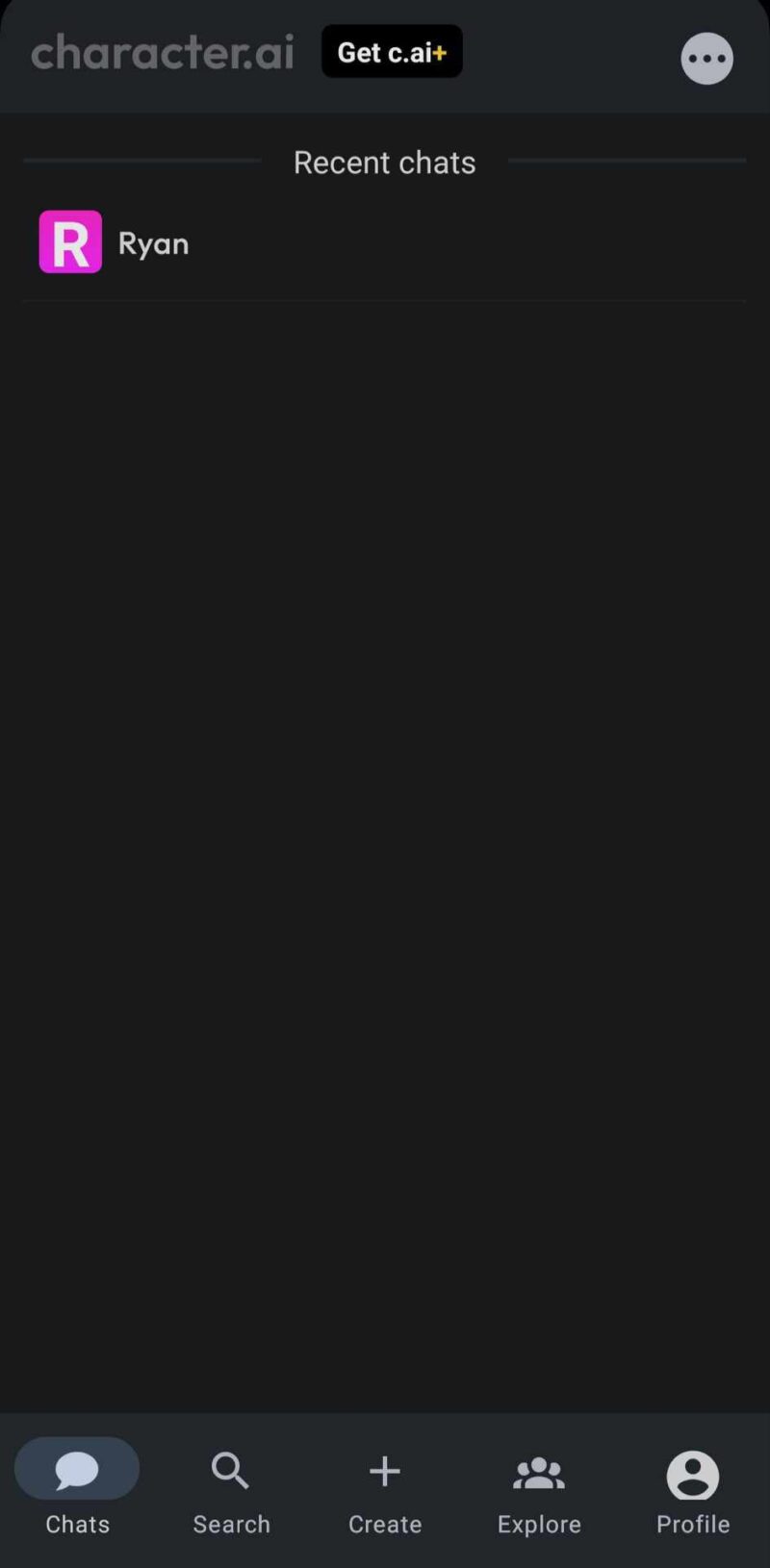The image has a black background with various user interface elements displayed. At the top, the text "Character.AI" is written in gray. To its right, within a black circle, is the text "Get C.AI" accompanied by a very small yellow diamond. Further right, there's a small gray circle containing three horizontal dots. Below this, the section is labeled "Recent Chats."

In the "Recent Chats" section, there is a pink square featuring an uppercase white "R," representing a contact named "Ryan." The rest of the background is blank and black.

At the bottom of the image, there is a navigation bar with multiple icons and text labels. From left to right, they are: a speech bubble icon labeled "Chats," a magnifying glass icon labeled "Search," a plus sign icon labeled "Create," a silhouette of a person labeled "Explore," and a gray circle with a silhouette of a person's head and shoulders labeled "Profile."

Every element is clearly separated and detailed against the black background, making each function distinctly recognizable.